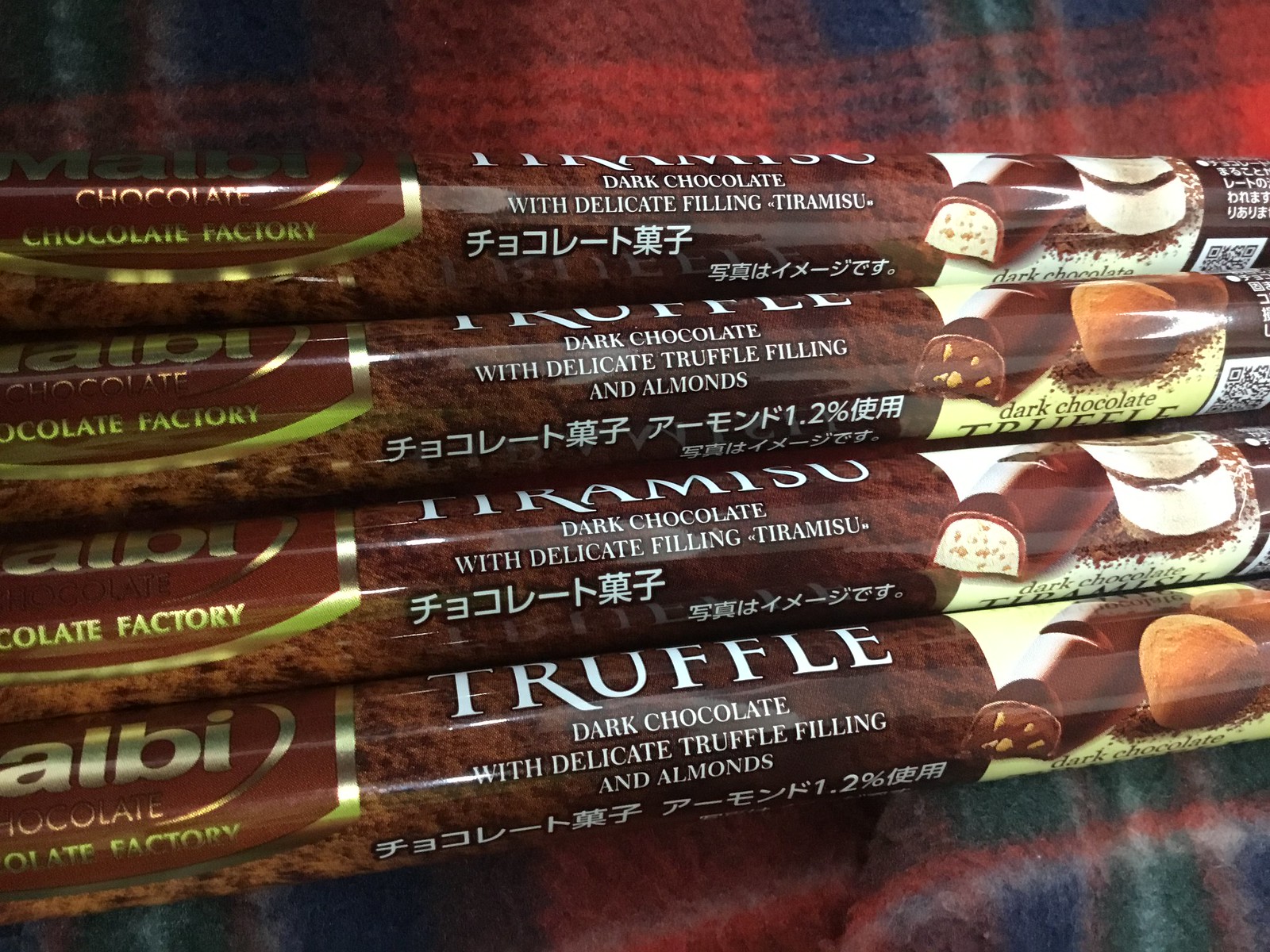This photograph captures four chocolate bar wrappers arranged vertically atop a red plaid fleece blanket with navy blue and white accents. Each wrapper prominently features the bold white text, "Truffle Dark Chocolate with Delicate Filling Tiramisu," accompanied by two lines of Japanese hiragana characters. To the right of the text, there are close-up images exhibiting the chocolate bars and their fillings, which range from creamy truffle to almond-studded variations. On the left side of each wrapper, the brand logo is displayed in metallic gold, outlined with bronze, partially readable as "Chocolate Factory." This sophisticated packaging sits harmoniously against the cozy background, highlighting the contrast between the luxurious treats and the soft, homey fabric beneath them.